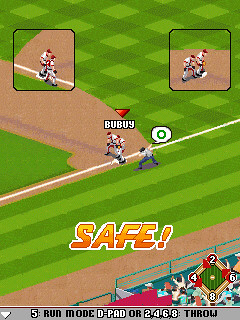This image is a detailed screenshot from a retro-style baseball video game reminiscent of the DOS era, evident from its basic, pixelated graphics and a color palette dominated by varying shades of green to illustrate the field. Dominating the center is a player, highlighted and labeled "B-U-B-U-Y," running diagonally along a white line. To his right stands an umpire, distinguishable by his white shirt, blue pants, blue hat, and black shoes, with a speech bubble above his head containing a green circle. Both of these central figures are situated near what appears to be first base.

In the upper left and right corners of the image, there are zoomed-in views of players positioned near bases, encased in black square outlines. These figures, in white jerseys with red hats and accents, are engaged in the game, further emphasizing the in-game action. One of the figures on the left is seen standing on third base, while the mirrored arrangement on the right reflects similar characteristics.

Marked prominently at the bottom center in bold orange-yellow text, the word "SAFE!" signals an in-game event, underscored by a white outline for emphasis. Below this, a gray banner provides gameplay instructions: "5: Run Mode D-Pad or 2, 4, 6, 8: Throw." To the bottom right, a schematic of the baseball field is presented with bases numbered 2, 4, 6, and 8, overlaying a backdrop of fans seated in blue stands. This meticulous layout encapsulates the immersive yet simplistic charm of an era-defining sports video game.